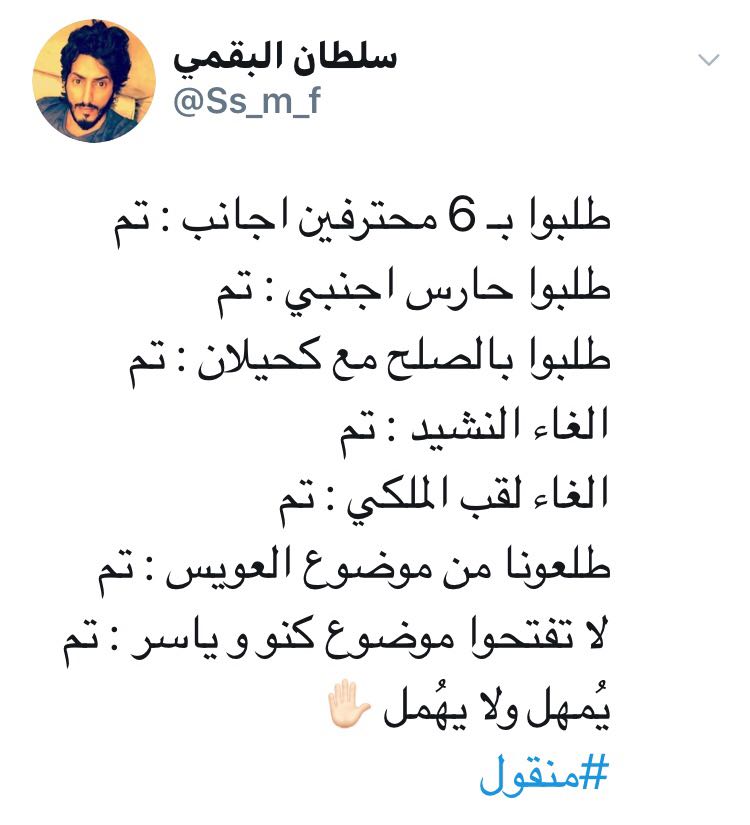The image is a screenshot of a social media post, likely from Twitter, displaying content in what appears to be Arabic script. In the top left corner, there's a small circular profile picture of a man with black hair, a black mustache, and beard. His hair is medium-length and curly, and he's wearing a blue shirt while standing against a yellow-orange background. To the right of the profile picture, the user's name and handle (@SS_M_F) are presented in black text. Below the username, there are eight lines of text in Arabic, with notable elements including the number six on the first line and a hand emoji at the very bottom. At the bottom of the text, there's a blue hashtag, though the exact wording is unclear.